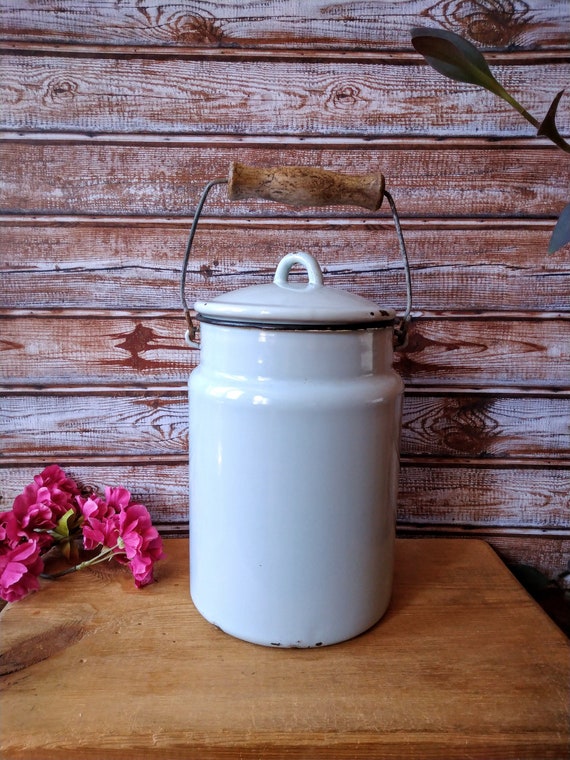The image depicts a close-up of an antique-style ceramic milk jug, featuring a glossy white cylindrical body with a few dents and slight rust. The jug has a metal band that arches over the top, connected to a wooden handle, which is facing upwards. This jug is equipped with a matching white ceramic lid that has a small arched handle in the center. The jug sits on a wooden table, contrasting with a rustic, knotty pine wood wall in the background, which displays grayish hues and highlighted brown knots, reminiscent of old barn wood. Lying next to the jug on the table is a purple flower, adding a touch of color to the scene, which is brightly lit with clear visibility.